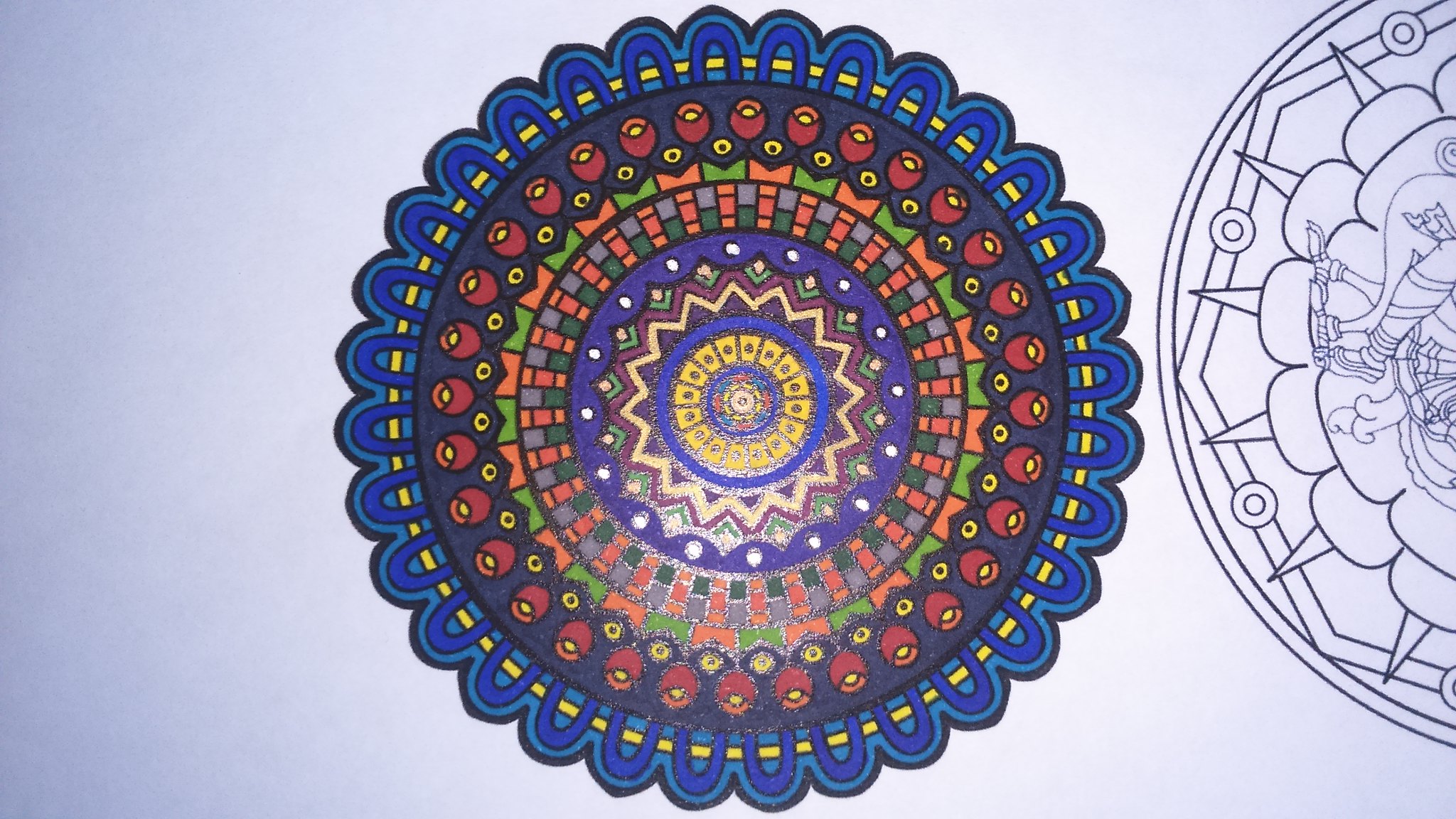A horizontal coloring page features intricate mandalas against a light gray to whitish backdrop. The detailed mandalas exhibit crest-like qualities, with rhythmic, round, and uniform design elements that exude a mystical aura. Dominating the focus, a fully colored mandala appears primarily in shades of blue. The outer edge of this mandala is adorned with upside-down U-shaped scalloping, outlined in a darker navy blue. Just inside this border, a vibrant yellow ring encircles the mandala's core.

Within this ring, there resides a full circle of flower buds interspersed with eye-shaped and bead-like figures, adding layers of intricate detail. Following this band is a checkered ring, enameled in a blend of pink, blue, and lavender hues. At the very center, a crest emerges with a sunburst pattern, highlighted by lavender, beige, and dark blue with beige accents, and a yellow core.

To the right, partially visible, is another mandala, this one uncolored. Embedded within its design appears to be a figure resembling a Greek character's foot in a sandal, which winds up the lower leg. Additionally, intricate elements suggestive of bird or horse legs are also woven into this incomplete mandala, adding to its enigmatic charm.